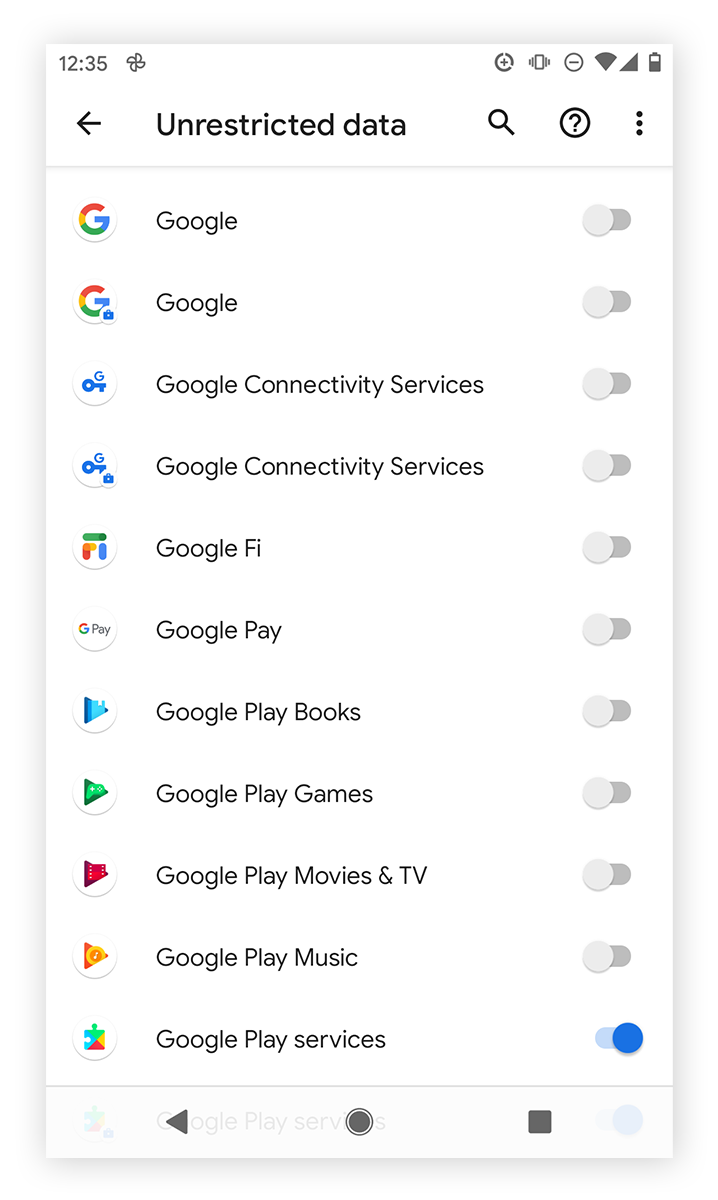This is a screenshot of an Android phone's settings page. The rectangular screen prominently displays the Google search engine's search bar, with the current time "12:35" shown in the top left corner. In the upper right corner, there are icons including a magnifying glass, a circled question mark, and a three-dot menu for additional options. 

In the search bar, the user has typed "Unrestricted Data" with a capital "U." Below the search bar, a list of various apps is visible, including Google, Google Play Books, Play Games, Play Movies & TV, and Play Music. Each app has a corresponding toggle bar to its right. All the toggle bars for these apps are in the "off" position, except for the toggle bar next to "Google Play services" at the bottom, which is switched "on."

At the very bottom of the screen, the navigation bar is visible, featuring a central home button flanked by a tab button on the right and a back button on the left. The overall layout suggests that the user is in the settings section of their phone, managing data usage permissions for different apps.